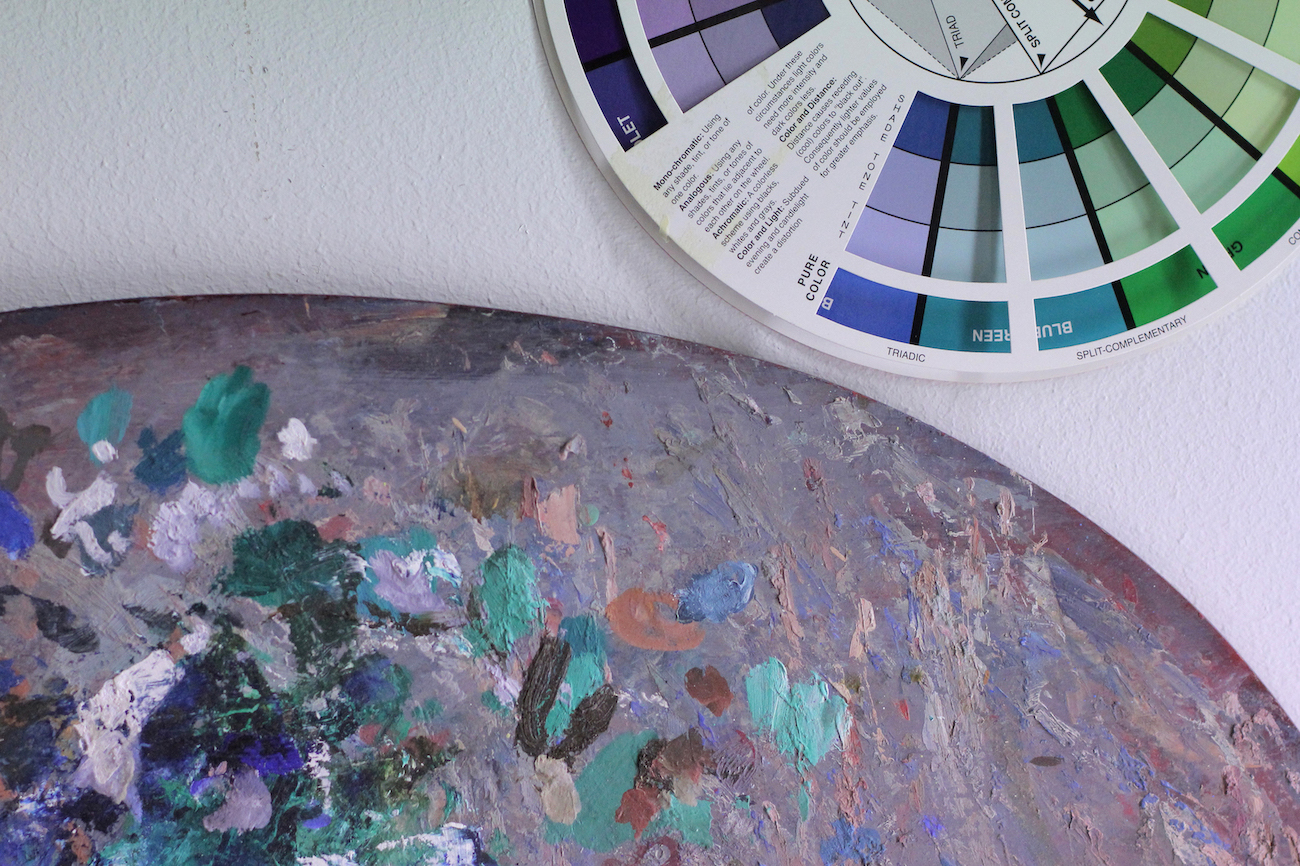This image provides a detailed, top-down view of a white-painted table supporting two primary objects. Dominating the bottom left of the image, there is a round ceramic or stone plate adorned with a myriad of paint swatches, predominantly teals, blues, and purples, suggesting the remnants of an artist’s palette. The plate features an abstract, possibly floral pattern consisting of greens, blues, and whites, hinting at artistic experimentation or a unique piece of artwork. On the top right, a color wheel for color theory is positioned, showcasing a spectrum of hues and corresponding shades, likely serving as a tool for the artist to choose and mix accurate colors. The overall arrangement, with the color wheel and painted plate on a clean, white surface, evokes a scene of artistic creation and planning.